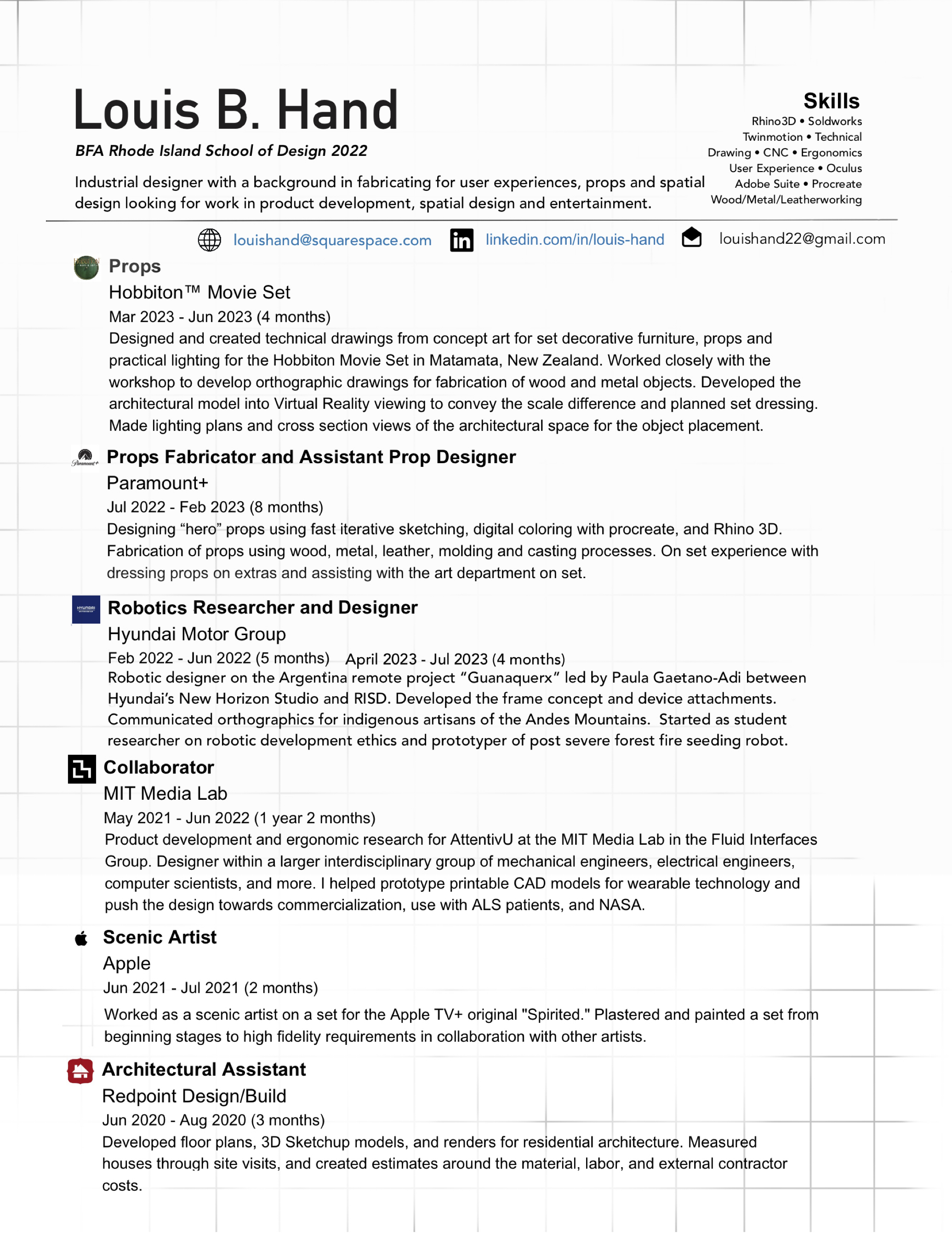The image captures a detailed resume of Lewis B. Hand, BFA, a 2022 graduate of the Rhode Island School of Design. The resume is presented on a white background with black text and framed within black squares. At the top, Lewis's name is prominently displayed, followed by a brief paragraph describing him as an industrial designer with a background in fabricating for user experiences, props, and spatial design, seeking positions in product development, spatial design, and entertainment.

To the right, a list of skills is partially visible, showcasing abilities in technical drawing, CNC, ergonomics, user experience, Oculus, Adobe Suite, and various forms of craftsmanship including wood, metal, and leatherworking. Below this section are hyperlinks to his Squarespace, LinkedIn, and Gmail addresses.

Beneath this introductory section, the resume is segmented into detailed accounts of Lewis's work experience, each accompanied by small iconographic images and descriptive paragraphs:

1. **Props, Hobbiton Movie Set (March 2023 - June 2023, 4 months):** Designed and created technical drawings for set decor, props, and lighting for the Hobbiton movie set in Matamata, New Zealand. Collaborated closely with the workshop to produce orthographic drawings for wood and metal fabrications and developed virtual reality models for spatial planning.

2. **Props Fabricator and Assistant Prop Designer, Paramount+ (July 2022 - February 2023, 8 months):** Designed "hero props" using iterative sketching and 3D modeling software, and fabricated props using various materials. Gained on-set experience dressing props and assisting the art department.

3. **Robotics Researcher and Designer, Hyundai Motor Group (Two periods: February 2022 - June 2022 and April 2023 - July 2023, totaling 9 months):** Worked on the Argentina remote project Guanacorx, developing frame concepts and device attachments, and provided orthographic communications for indigenous artisans. Conducted ethical research and prototyping for post-forest fire seeding robots.

4. **Collaborator, MIT Media Lab (May 2021 - June 2022, 1 year 2 months):** Contributed to product development and ergonomic research for Attentive View at MIT's Fluid Interfaces Group. Participated in prototyping wearable technology for ALS patients and NASA, working with a multidisciplinary team.

5. **Scenic Artist, Apple (June 2021 - July 2021, 2 months):** Worked on Apple TV+ original, Spirited, plastering and painting sets to meet high visual fidelity standards in collaboration with other scenic artists.

6. **Architectural Assistant, Redpoint Design/Build (June 2020 - August 2020, 3 months):** Developed floor plans, 3D models, and renders for residential projects, conducted site measurements, and created material and labor cost estimates.

The resume's structured layout and detailed descriptions of Lewis's varied experience highlight his comprehensive skills and specific contributions to each project, envisaging a well-rounded and capable industrial designer poised for future opportunities in his field.